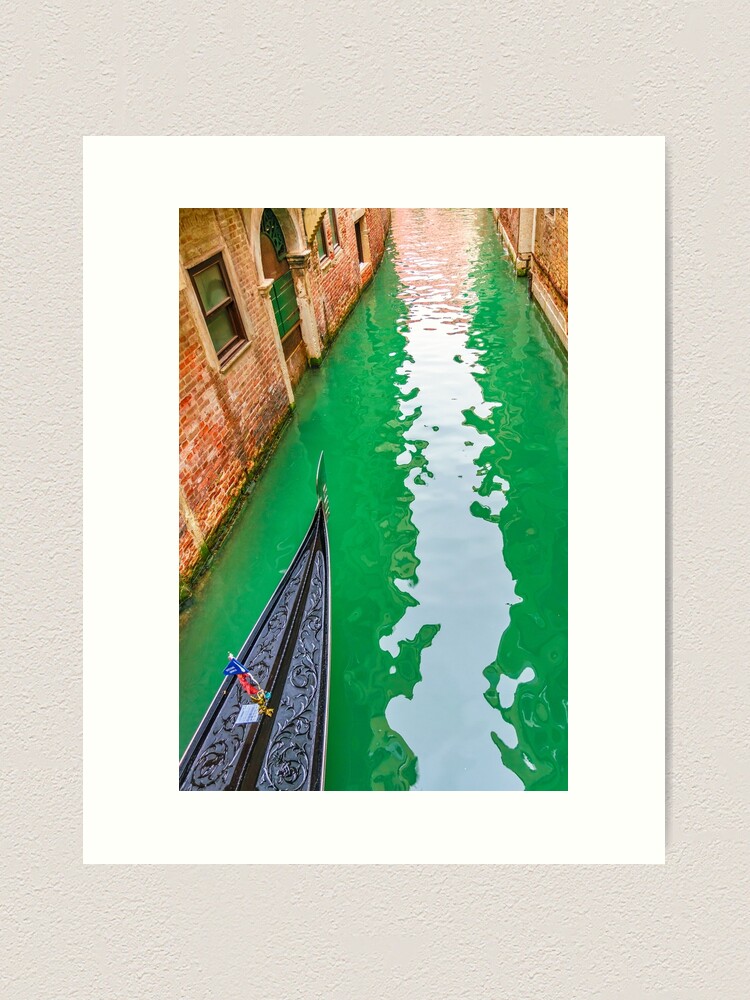This framed aerial photograph, mounted on a white canvas and displayed on a white wall, captures a picturesque waterway in Venice. The shot showcases the deep, brilliant green water of the canal flanked by two ornate, red brick buildings adorned with windows and archways. Sunlight bathes the scene, illuminating the center of the canal where the water's color subtly shifts. At the lower left corner of the image, the narrow, ornate, pointed tip of a blue gondola enters the frame, suggesting movement through this tranquil passageway. The photograph's lighting is bright and clear, highlighting the rich textures and vivid colors of this Venetian setting.